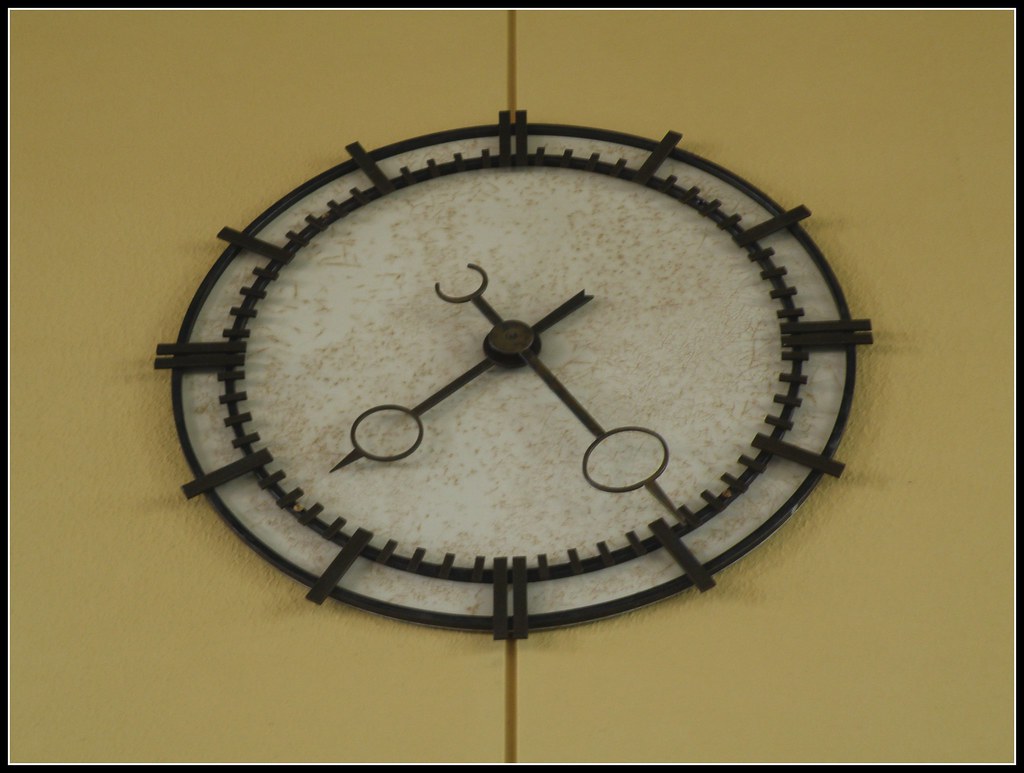The image features a minimalist clock face without numerical markings, set against a beige-yellow background. At the center of the clock, there is a circular area with a white backdrop. Two metallic clock hands are positioned in the middle, each designed with pointed tips and small circular accents near these tips. Radiating outward from the clock center are several vertical lines, arranged as if to denote the positions where numbers would typically appear on a traditional clock face. The overall design is both simple and elegant, emphasizing the passage of time through clean lines and understated aesthetics.